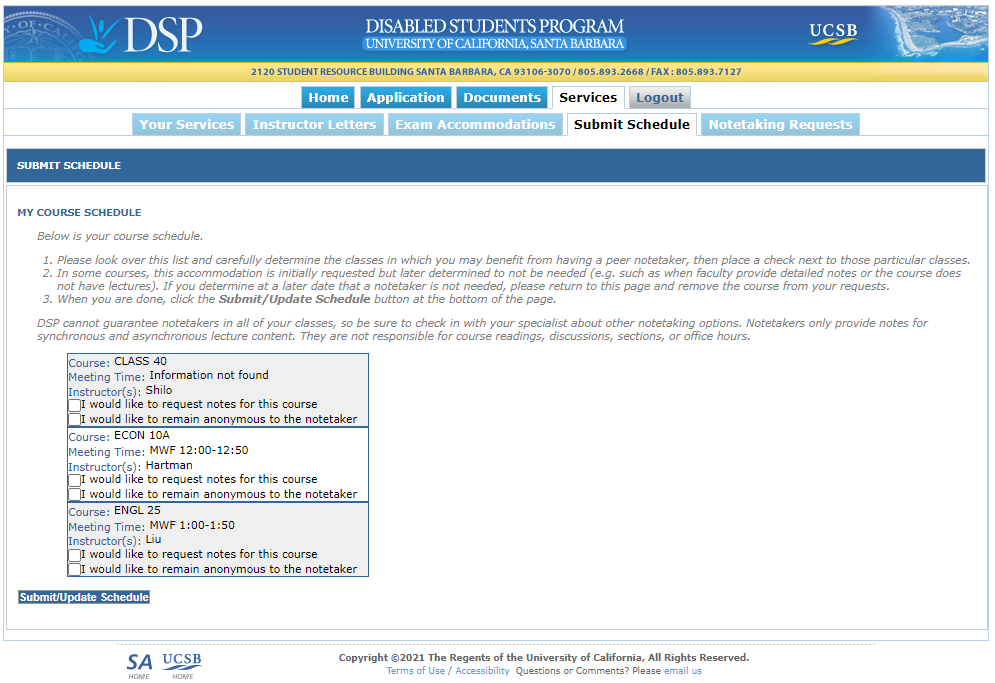This image depicts a section of the University of California, Santa Barbara's Disabled Students Program (DSP) website. At the very top center, the title "Disabled Students Program" is prominently displayed in white text. Directly beneath this, the text "University of California, Santa Barbara" is also in white, but set against a light blue rectangular background. In the top right corner, the abbreviation "UCSB" is shown, while the top left corner features "DSP" along with a logo illustrating a hand holding a person.

Just below these elements, a thin yellow strip provides the contact information: "2120 Student Resource Building, Santa Barbara, California 93106-3070." Underneath this, the website's navigation bar is divided into five primary sections: Home, Applications, Document, Services, and Logout. Additionally, there are five more specialized sections for registered users: Your Services, Instructor Letters, Exam Accommodations, Submit Schedule, and Notetaking Requests.

Towards the bottom left of the image, there are three small labeled boxes representing different classes: "Class 40," "Econ 10-A," and "ENGL 25."